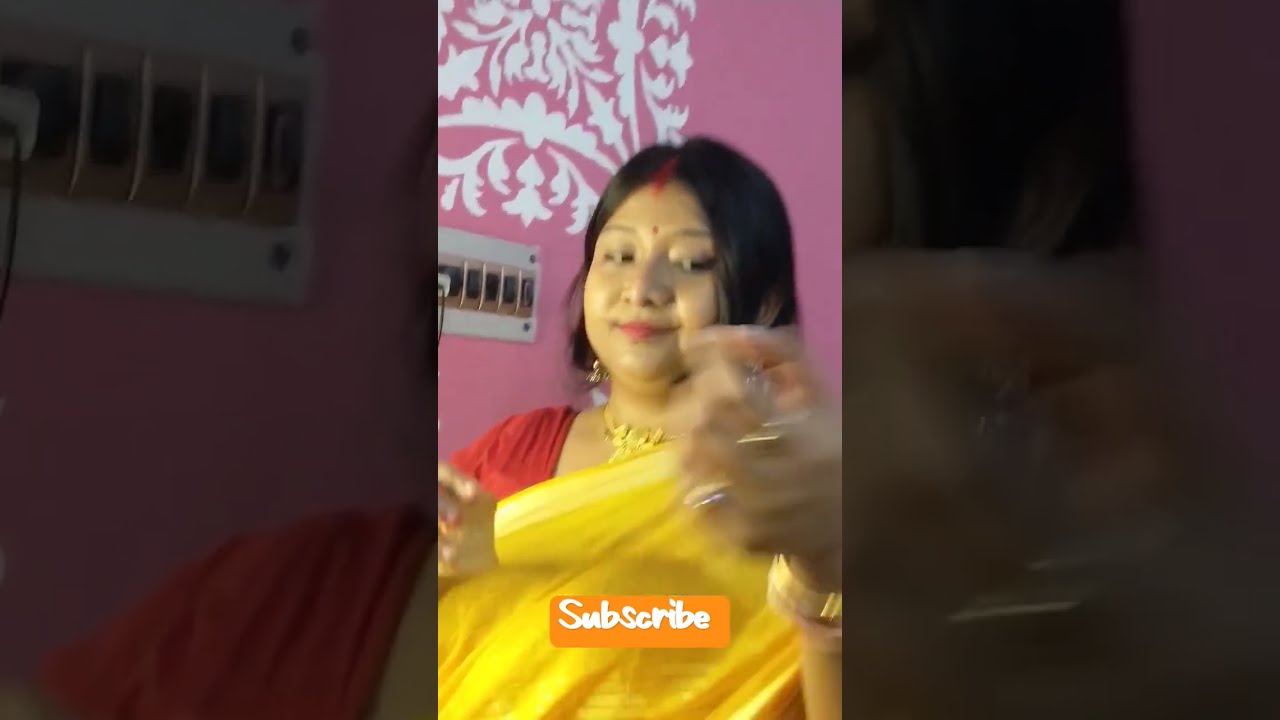The image is a screen capture from a social media video, likely TikTok, filmed in portrait orientation and recorded on a phone. The screen has been cropped, making the sides significantly longer than the top and bottom, with a zoomed-in effect. An orange rectangle overlay at the bottom of the screen features the word “subscribe” in white Comic Sans font.

Central to the image is an Indian woman visible from her mid-torso upwards, adorned in traditional attire. She wears a short-sleeve reddish-orange dress paired with a yellow sari draped over her shoulder. Her accessories include a red dot (bindi) on her forehead, a gold necklace, dangling gold earrings, multiple gold bracelets on both arms, and several gold rings on her fingers. She has straight, dark brownish-black hair that falls just above her shoulders. One of her arms is raised, and her hand is in motion, pointing towards the camera and creating a slight motion blur.

The backdrop is a pink wall with an intricate white floral pattern, adding a decorative element to the scene. The overall composition suggests dynamic activity, capturing a candid moment from the video.